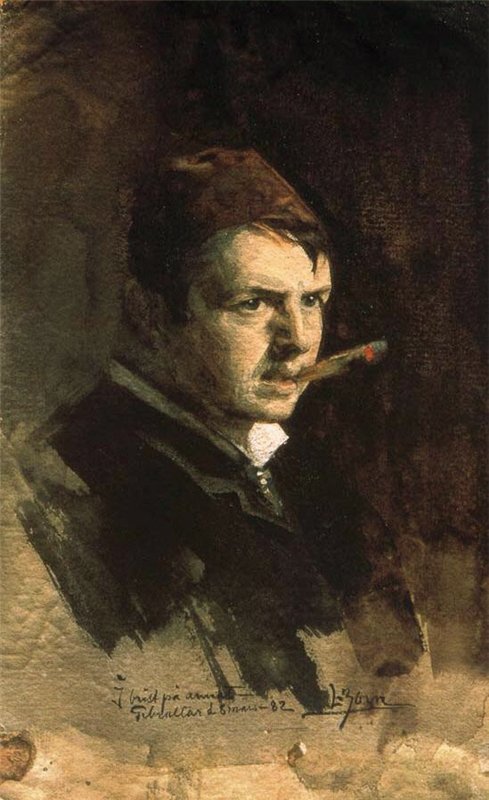The image is a detailed, vintage painting, likely an oil or watercolor, depicting an older man in historical attire. The man, who is clean-shaven and white, is centrally positioned in the painting, gazing to the right with short dark brown hair and brown eyes. He is dressed in a black suit with a white shirt underneath and has a lit cigar hanging vertically from his mouth. The background of the painting transitions from dark brown behind the man's head to lighter sandy and greenish shades below. The overall style reflects an older, perhaps early 20th-century, artistic approach. At the bottom of the painting, there is a handwritten signature or description, possibly in a different language, which includes phrases like "J. Brist, P.A. Annetre, Gabriel Tarr, Sinaris 82," and some indistinct letters and numbers, suggesting the names of individuals or an additional context related to the artwork.